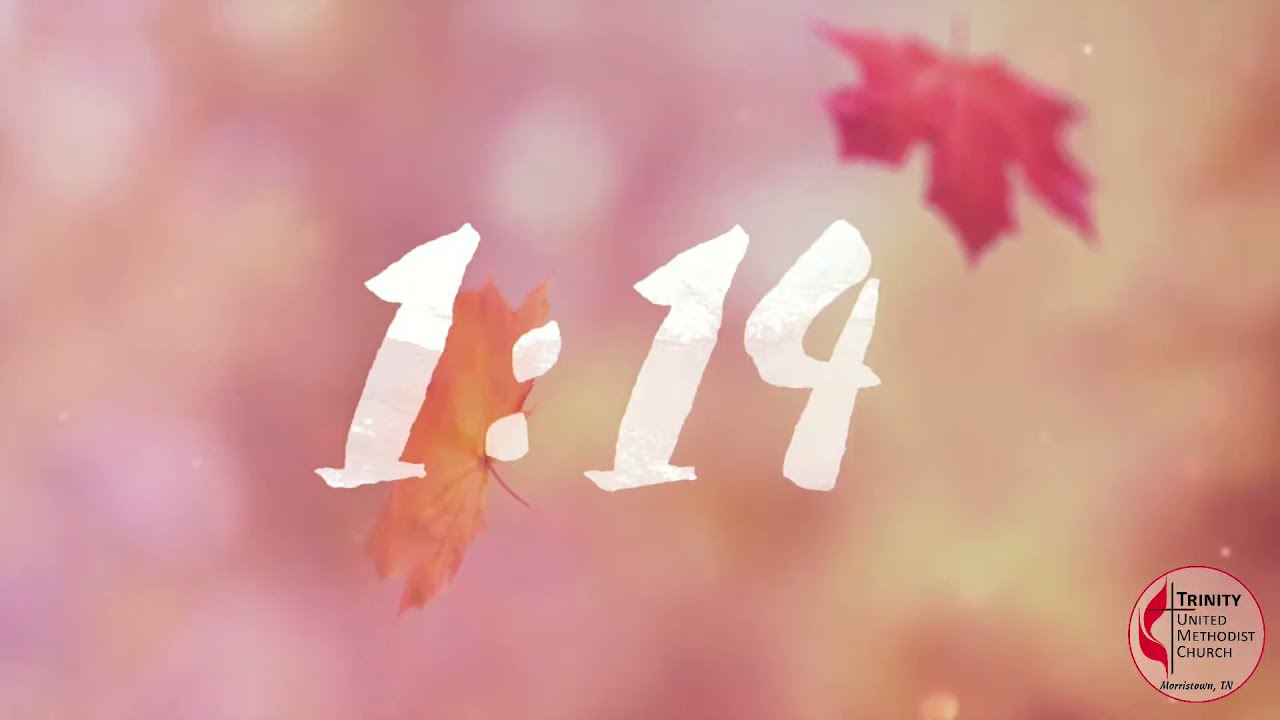This image features a beautifully blended watercolor background in shades of pink, peach, yellow, and red. In the center, the time "1:14" is printed in white with a brushstroke effect, suggesting the appearance of watercolor. Overlaying this background are two distinct maple leaves: one, a red leaf positioned near the top right corner and turned upside down, and the other, a golden-orange leaf behind the number "1" in the time display. Additionally, the bottom right of the image includes a circular emblem with a red border, containing the text "Trinity United Methodist Church, Morristown, Tennessee," with "Trinity" in bold, capitalized letters. The emblem also features a red two-flame logo behind a cross.